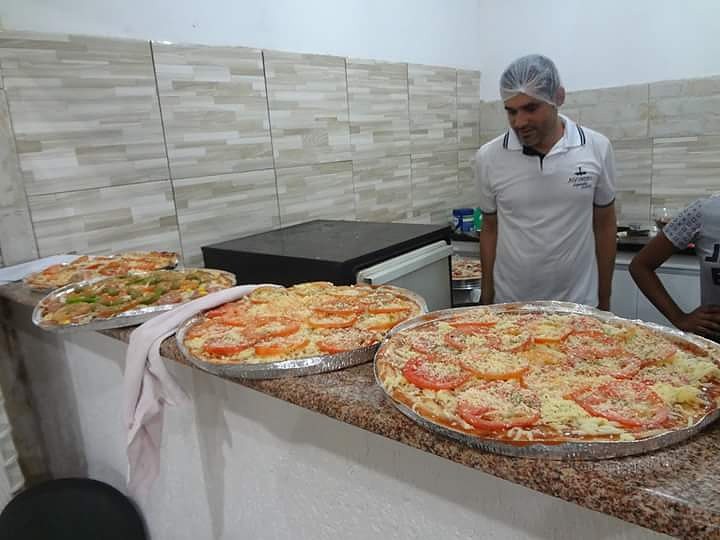The photograph captures a detailed, bustling scene inside a restaurant from a customer's perspective at the front counter. Central to the image is a man, presumably the chef, identifiable by his white polo shirt adorned with an illegible logo on the upper left chest and a secure white hairnet. He is standing behind a counter filled with four large pizzas, each resting in thin, round tin pie pans. The pizzas, arrayed on a shelf, display a variety of toppings: the two closest to the viewer boast large tomato slices and generous amounts of cheese, while one of the more distant ones features prominent green pieces. The image is angled from the right side, tapering toward the left where the counter meets the wall, making the counter appear narrower in that direction. Only the arm of a second person is visible next to the chef, suggesting another presence without revealing their full identity. The restaurant's white wall and a blurry assortment of background objects complete the busy yet focused scene, emphasizing the chef's concentration on the array of pizzas.